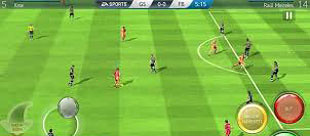The image depicts a football (soccer) game being played on a mobile phone, evident from the joystick controls displayed on the bottom corners of the screen. The game interface prominently features EA Sports branding, suggesting it could be an older version of FIFA. There are two team scorecards at the top, showing the scores and remaining time, with one team identified as Real Madrid. Players on the field wear black and white or red and white kits, and the green field is detailed with alternating lighter and darker stripes, white lines, and a semicircle on the right side. The control scheme includes a silver joystick for navigation on the left, and red, yellow, and green buttons on the right. Despite being very small and somewhat blurry, the image clearly captures the essence of an old-school mobile football game with accurate in-game elements and controls.